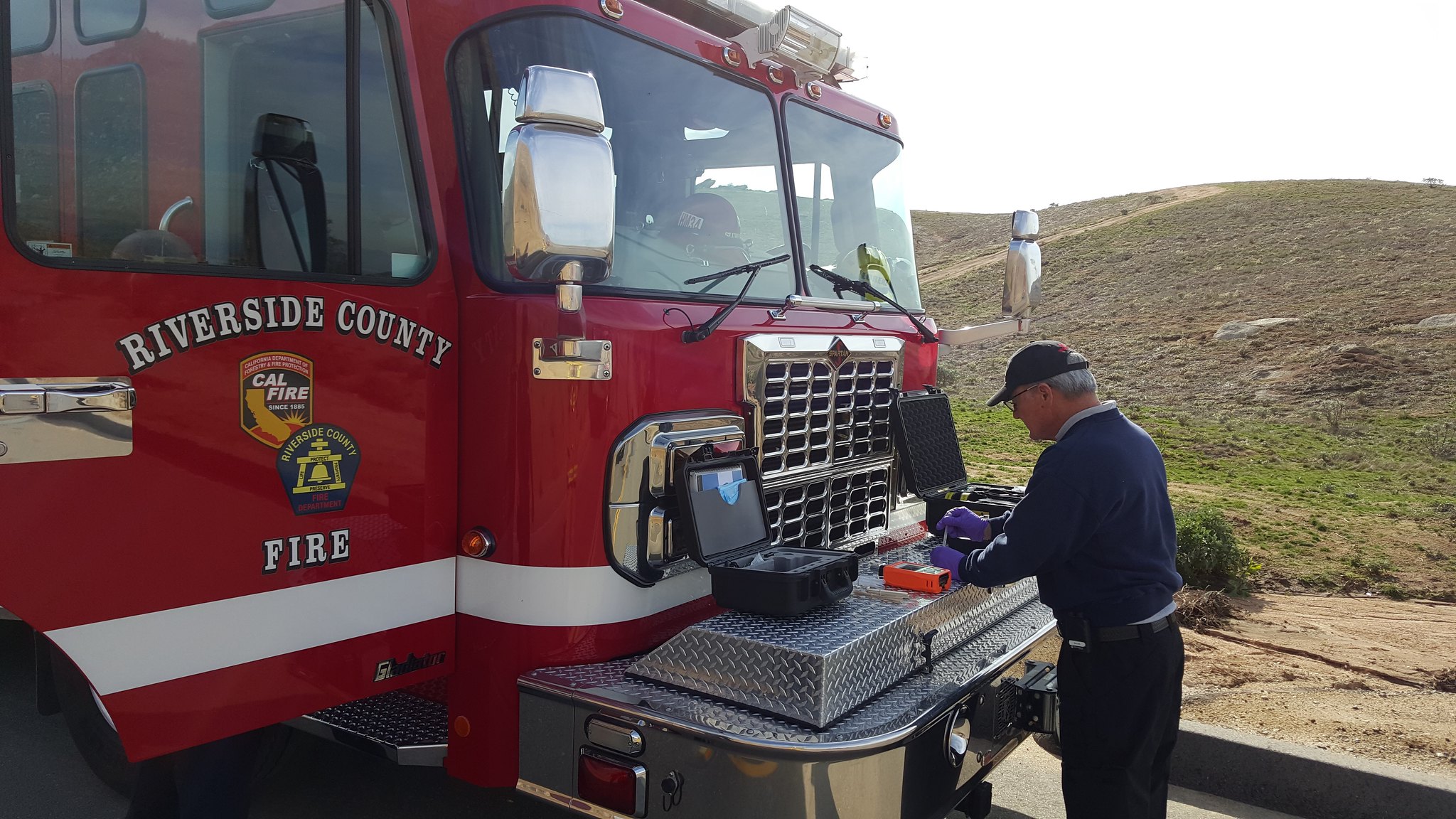A silver-haired man wearing a navy blue sweatshirt, black pants, a blue cap, and purple gloves is standing in front of a Riverside County fire truck. The fire truck's door is open, displaying the "Riverside County Fire" text along with a Cal Fire logo and another county logo. The front of the fire truck features a wide bumper that the man is using as a makeshift workstation. He has two open toolboxes and is working with a small screwdriver or similar tool, possibly handling some liquid instrumentation. In the background, there are low, mostly brown hills with sparse green grass, indicating a potentially cloudy or overcast day as the sky appears white.